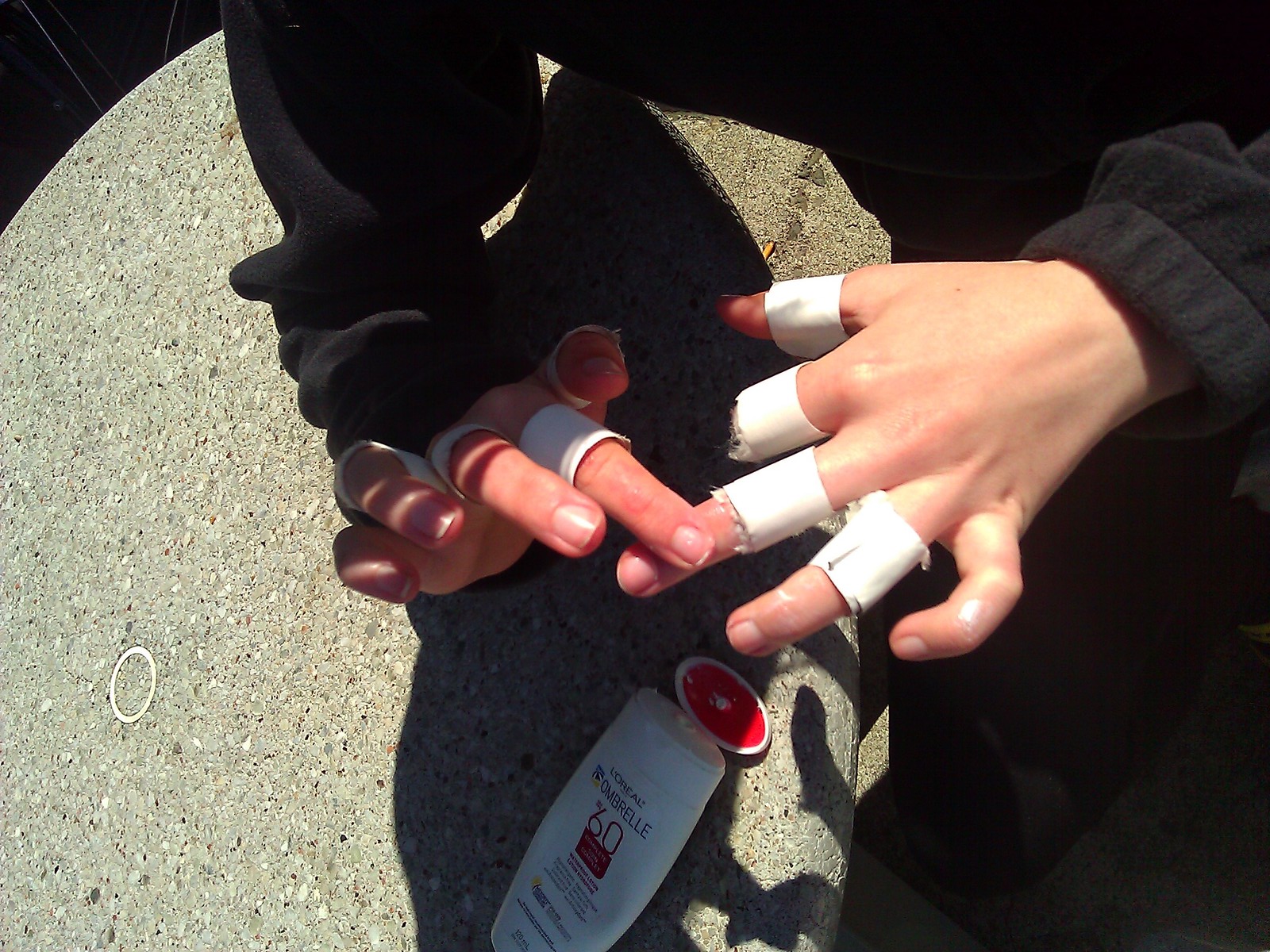An outdoor color photograph taken in bright sunlight centers on the hands and forearms of a Caucasian individual, potentially a teenager. Both hands are prominently featured, with the left hand, palm down, displaying fingers extended. White bandages are wrapped below the first knuckle on the thumb, index, middle, and ring fingers, but not the pinky. The right hand, partially in frame, has similar bandages and is positioned with fingers slightly bent. The person is wearing a black sweater and appears to be standing near a concrete surface that includes a brass circle, which could be a decorative element or functional feature like a water source. A bottle of lotion with orange lettering reading "60" lies nearby, indicating the person is likely applying lotion to their fingers. Additionally, there is a shadow on the ground with a ribbon bearing a readable number "60," adding to the scene's detailed context.